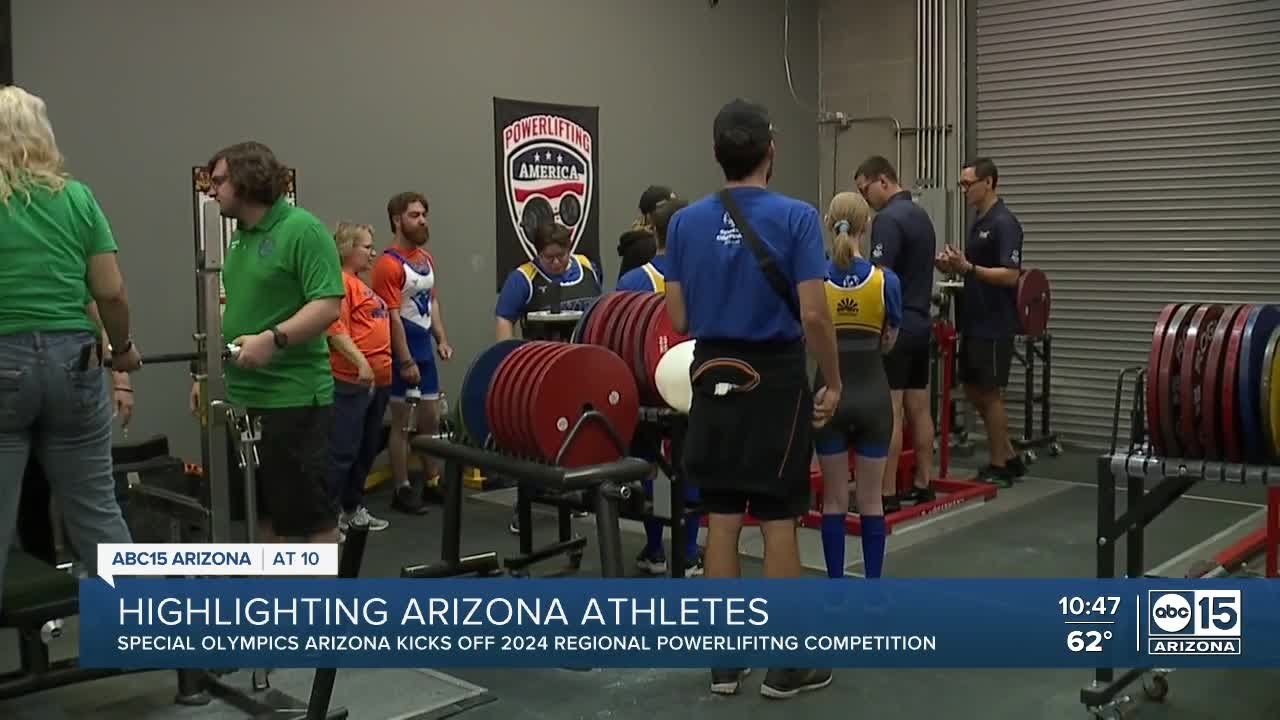The image is a still from an Arizona-based news channel, ABC 15, highlighting the Special Olympics Arizona as they kick off the 2024 Regional Powerlifting Competition. The bottom of the screen features a blue rectangular label with the text: "Highlighting Arizona Athletes, Special Olympics Arizona Kicks Off 2024 Regional Powerlifting Competition," alongside the ABC 15 Arizona logo and a temperature reading of 62 degrees. The scene is set in what appears to be a weightlifting room, possibly part of a warehouse or a large garage, indicated by a distinctive garage-style door in the upper right-hand corner.

In the room, numerous weights are organized on stands, with the majority being red, and a few in blue and green. Around 12 to 15 individuals are present, including both men and women. Some of them are wearing weightlifting gear, indicating they are competitors, while others are dressed in green T-shirts and jeans or black sports shorts and navy shirts, suggesting they might be volunteers or spotters. The background features a partially visible poster that reads "Powerlifting America." The atmosphere suggests that preparations are underway for the competition to begin.